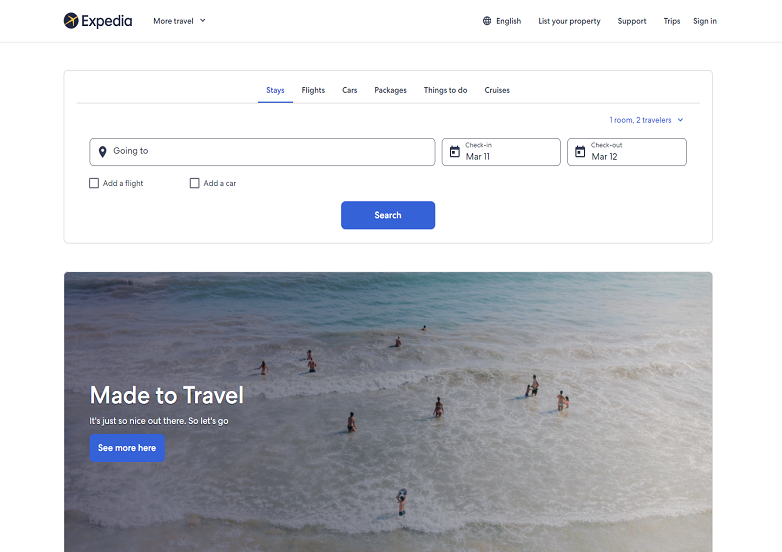This image, sourced from the Expedia website, showcases the interface prominently featuring the Expedia branding on the upper left-hand side. The brand name "Expedia" is displayed in black font with a capital "E," accompanied by a logo to its left—a black circle encompassing the thin outline of an airplane.

Adjacent to the logo, the top navigation bar includes a "More Travel" dropdown menu, followed by several action buttons aligned to the right: "English," "List Your Property," "Support," "Trips," and "Sign In." A thin separator line demarcates this navigation section from the interactive search area below.

The central interactive section features a search box labeled "Going To," flanked by "Check-in" and "Check-out" boxes, facilitating travel bookings. Above this search bar is a horizontal menu offering various travel options: "Stays" (selected by default), "Flights," "Cars," "Packages," "Things to Do," and "Cruises."

Further down, an inviting, vibrant image captures the essence of travel—aerial view of people swimming in a crystal-clear ocean, embodying a sense of adventure and relaxation. Overlaying the picture is an inspiring slogan "Made to Travel," accompanied by two interactive buttons: a prominent blue "See More Hair" button, inviting users to explore additional options and a secondary "Same Hair" button offering more specifics. 

Overall, this layout not only prioritizes user navigation but also entices potential travelers with striking visuals and an intuitive interface.